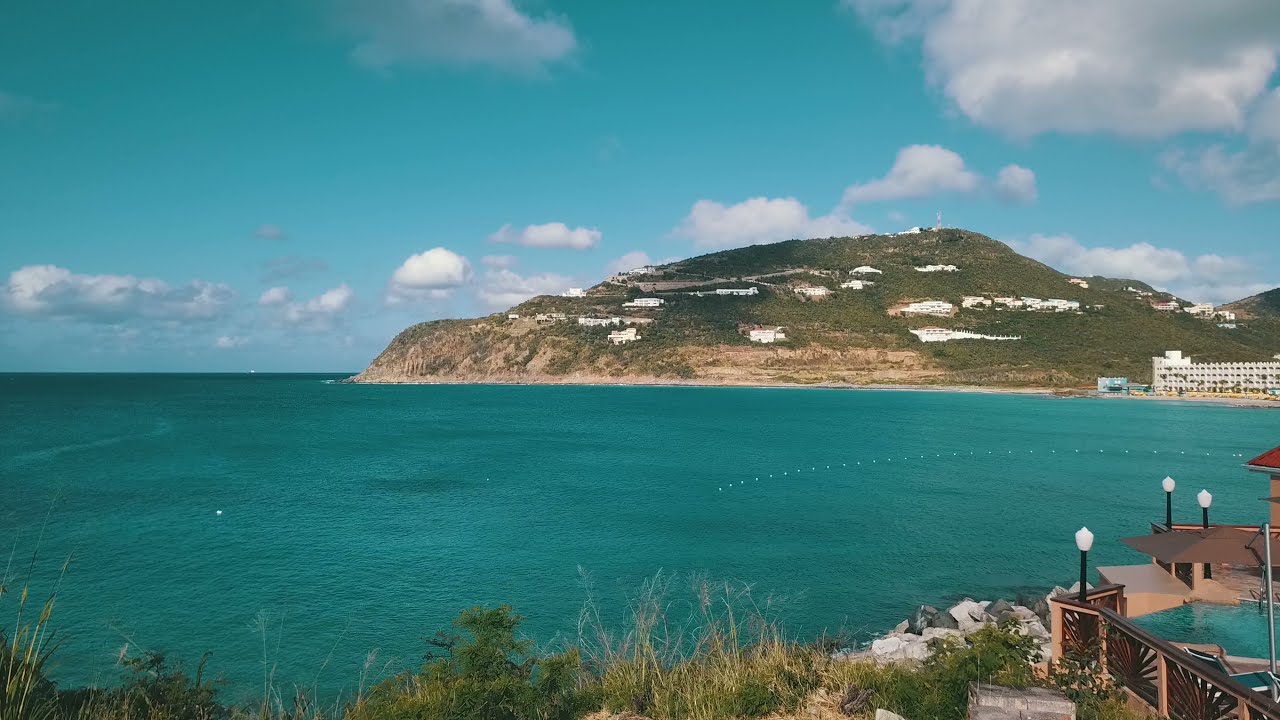The photograph captures a serene oceanside scene, where the turquoise and bluish-green waters stretch across the middle of the image. Along the bottom edge of the photo, sparse tall grass and weeds intermingle with the rocky shore. In the bottom right corner, a partial view of a gazebo-like structure and the corner of an outdoor pool is visible next to a barrier featuring three lampposts, suggestive of a lighthouse precinct.

Dominating the background, a landmass with gentle, hill-like contours extends into the ocean, creating the impression of a peninsula marking the entrance to a bay. This hill is adorned with white houses and other buildings, while greenery and rocky patches cover its slopes. Above, the sky spans a light blue hue, harmonizing with the sea’s color and interspersed with scattered clouds.